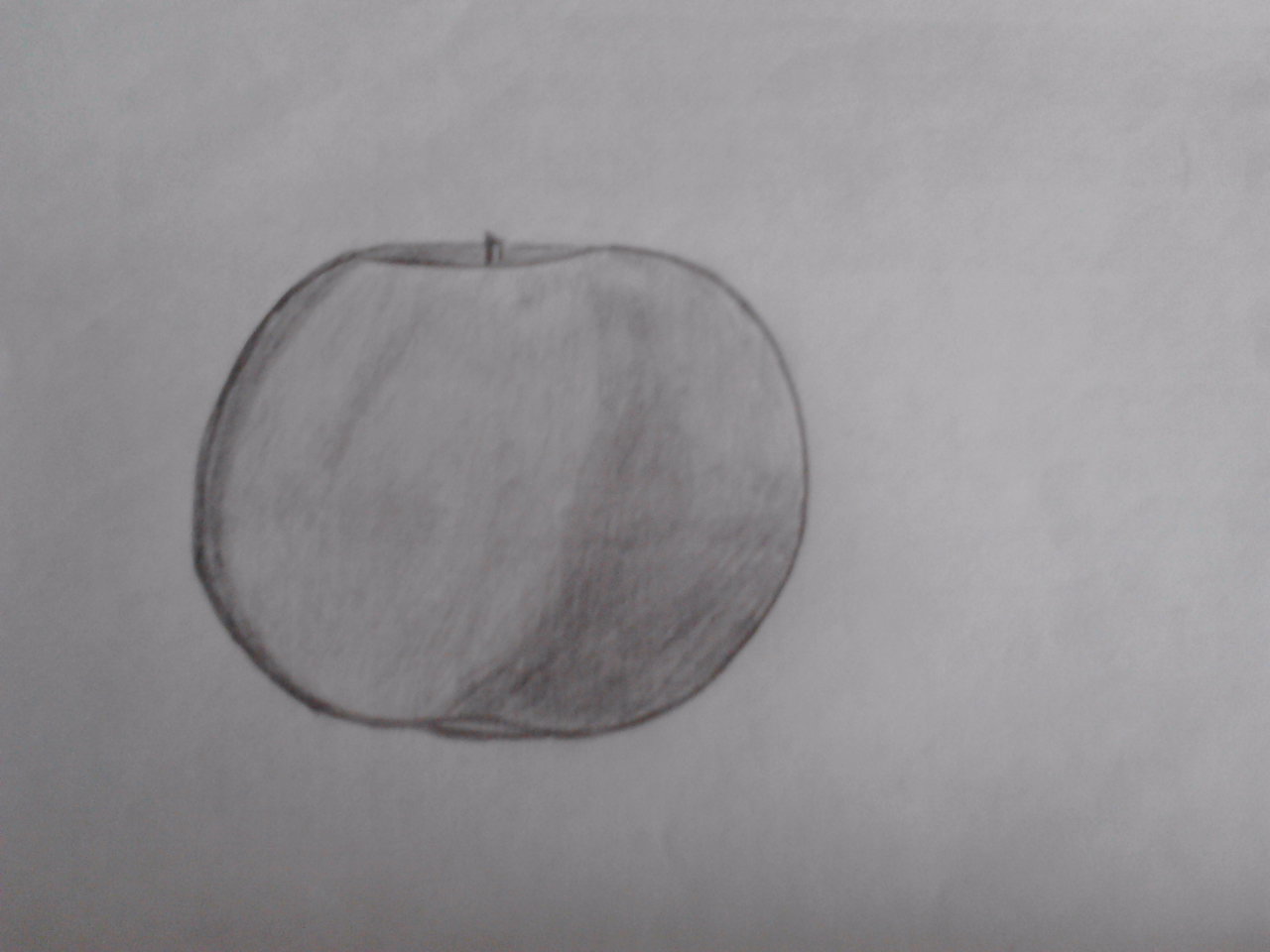This black and white photograph features a minimalist line drawing of an apple, set against a uniform grey background. The textured paper shows visible indents near the top, adding a tactile quality. Positioned off-center, the apple occupies approximately half the height and a third of the width of the image. The apple is predominantly round with a diminutive stalk emerging from the top. The right side of the apple is heavily shaded with dark pencil, while the left side exhibits lighter pencil strokes, adding a subtle gradation. More intense shading is visible along the left edge, contributing to a sense of depth and dimension. An additional indent near the top around the stalk enhances the 3D effect. A slight overlap at the bottom further accentuates the apple's dimensionality.